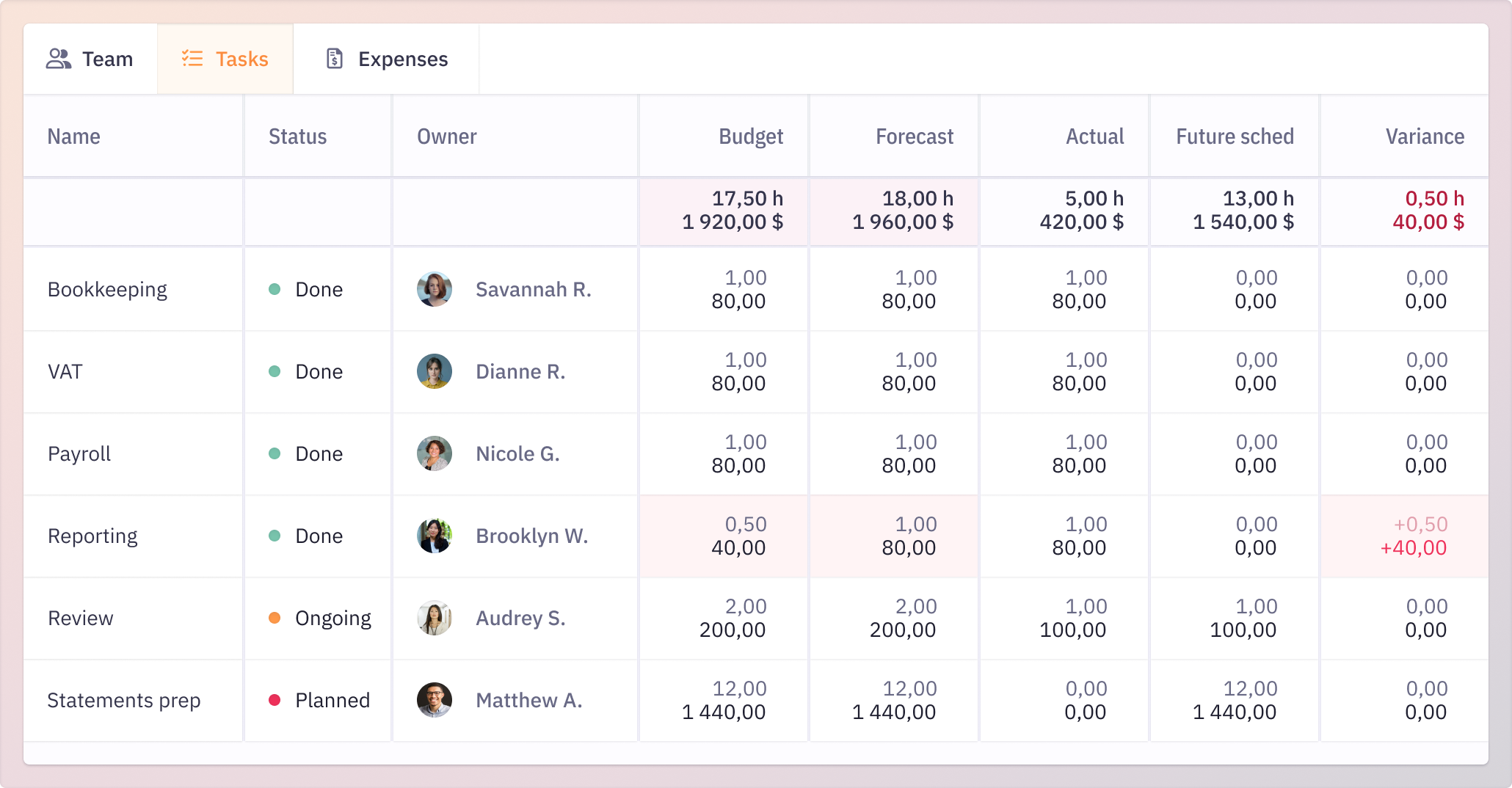This screenshot showcases a user interface with a light pink and gray color scheme. The interface features three primary tabs at the top: "Team," "Tasks," and "Expenses." The "Expenses" tab is highlighted, indicating it is currently selected.

The interface is divided into eight categories displayed in a tabular format: 
1. **Name**: The tasks listed under this category include Bookkeeping, VAT, Payroll, Reporting, Review, and Statement Prep.
2. **Status**: This indicates the completion status of each task. For instance, the Bookkeeping task is marked as "Done."
3. **Owner**: Shows the owner of the task, represented by an icon and a name. The owner of the Bookkeeping task is identified as Savannah R.
4. **Budget**: Displays the budgeted time and cost for each task. For Bookkeeping, it reads "1 hour, $80."
5. **Forecast**: Shows the estimated time and cost for task completion, identical to the budget for Bookkeeping at "1 hour, $80."
6. **Actual**: Records the actual time and cost spent on the task, which matches the budget and forecast for Bookkeeping at "1 hour, $80."
7. **Future Schedule**: Indicates upcoming planned time and cost, noted as "0 & 0" for Bookkeeping.
8. **Variance**: Shows any deviations from the budget and forecast, with no variance reported for Bookkeeping as it shows "0 & 0."

The owners of the tasks include:
- Savannah R.
- Diane R.
- Nicole G.
- Brooklyn W.
- Audrey S.
- Matthew A.

Icons to the left of these names suggest their identities, and all depicted individuals appear to be either white or light-skinned.